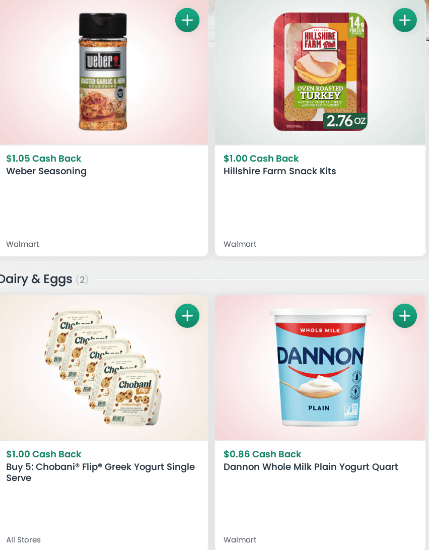This image appears to be a screenshot of a food shopping website featuring four product selections. Each product image has a green circle with a white plus sign in the top-right corner, indicating the option to add the item to the cart. 

1. **Weber's Seasoning**: The first product is displayed against a pink faded background showcasing a bottle of Weber's seasoning. The text indicates "105 cash back," and the product is available at Walmart, highlighted within a white area at the bottom.

2. **Hillshire Farm Snack Kits**: The second product shows a turkey snack kit with a gray background. The text on the image states "2.76 ounces" with the background in green and "$1 cash back" on the bottom right corner.

3. **Chobani Greek Yogurt**: The third product features the dairy and egg section, specifically Chobani Greek yogurt. The offer details "a dollar cash back" for purchasing five Chobani Flip Greek Yogurt single-serve cups. "All stores" is mentioned at the bottom left of this selection.

4. **Dannon Yogurt**: The fourth product is Dannon yogurt, shown against a pink faded background. The text includes "plain" flavor with the Dannon logo in light blue, and the word "Dannon" in dark blue. The cashback offer listed is "85 cents cash back."

Each product image and detail are organized to assist users in making informed purchasing decisions with cashback incentives prominently displayed.